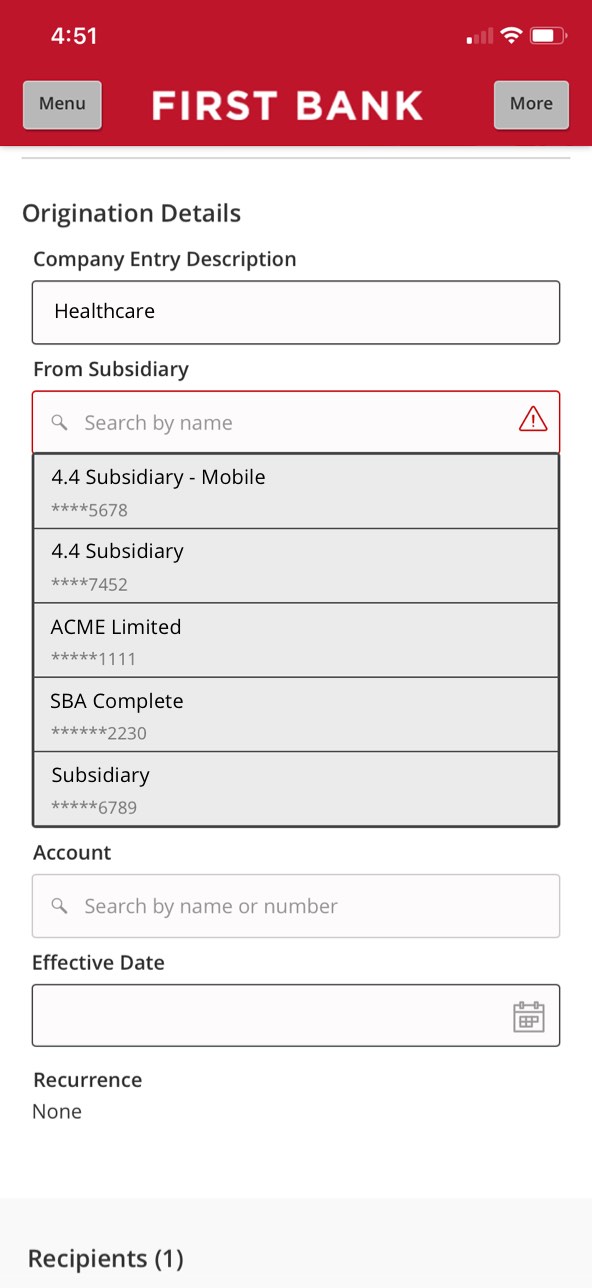Mobile Screen Capture of First Bank App Displaying Transaction Details

The screen capture, taken at 4:51, shows a mobile banking app interface from First Bank. In the top-right corner, indicators for signal strength, Wi-Fi strength, and battery life (approximately 75% full) are visible. The app features a red header background with "FIRST BANK" prominently displayed in large, white, capital letters. Flanking this title are two gray, rounded rectangular buttons with darker gray text; the left button is labeled "Menu" and the right button, "More."

Below the header, there appears to be a transaction table. The first row is labeled "Origination Details," "Company Entry Descriptions," "Healthcare," and "From Subsidiary." Each section acts as a header for the following entries. 

Within this structured table, multiple transactions are listed. A search text box, outlined in red, allows users to search by name. The account numbers within the transactions are partially censored with asterisks, revealing only the last four digits. Another header labeled "Account" includes a text box for searches by name or number. Adjacent sections include "Effective Date," which features a text box with a calendar icon likely used to select dates, and "Reoccurrence," which currently states "None."

At the bottom of the visible screen, a partially cut-off header labeled "Recipients (1)" is seen, but further details are not visible in the image.